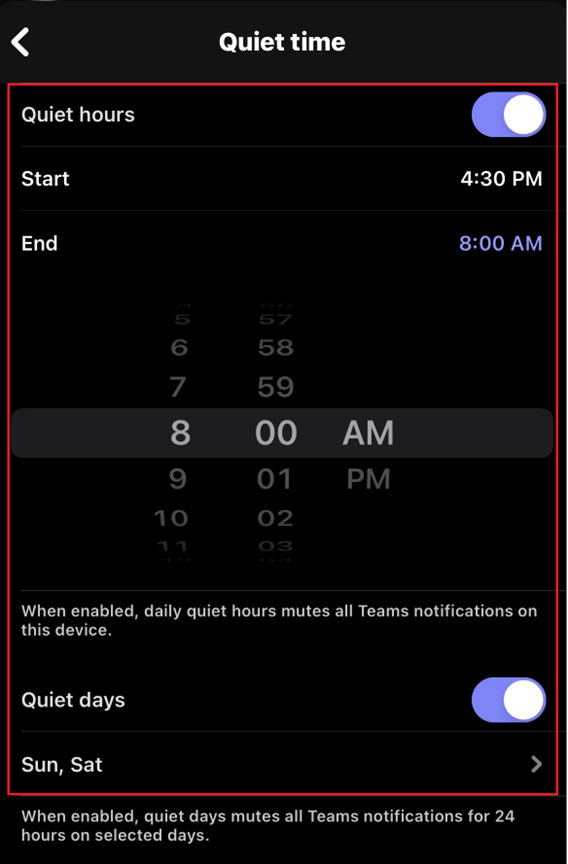This image depicts a cell phone screen displaying the settings for "Quiet Hours" within an application. The background is black. At the top, in bold white letters, it says "Quiet Time," enclosed within a red box. An arrow pointing to the left sits adjacent to "Quiet Time."

In the top left corner of the screen, there is another section labeled "Quiet Hours." Below this label is a toggle switch, which is currently turned on, indicated by a purple slider with a white circle. 

The settings show a start time of 4:30 PM and an end time of 8:00 AM. The start time is displayed in white font, while the end time is in purple. Beside these times are rotating numbers, resembling a clock interface, which allows users to adjust the times. The current display is set to 8:00 AM.

Below these time settings, the screen states: "When enabled, daily quiet hours mute all Teams notifications on this device." This text is presented in white print.

Further down, another option titled "Quiet Days" is visible, with a similar toggle switch turned on, indicated by the same purple slider and white circle. The specific quiet days are listed as Saturday and Sunday, with an arrow pointing to the right beside these days. 

At the very bottom of the screen, outside the red-outlined box containing all the settings, the text explains: "When enabled, quiet days mute all Teams notifications for 24 hours on selected days," also in white print.